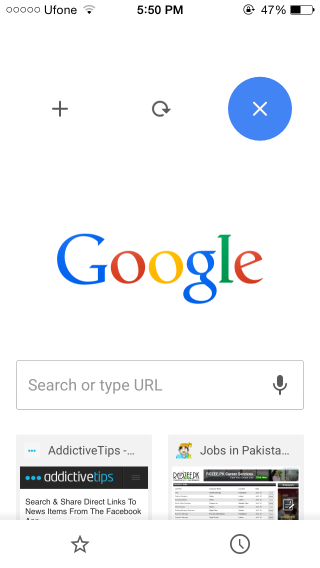A screenshot of a smartphone's browser interface is displayed against a white background. The status bar at the top indicates it is 5:50 PM, with icons for Wi-Fi, mobile signal strength, battery percentage at 47%, and other typical indicators including a lock within a circle and an arrow. 

Below the status bar, the Google search bar is prominently placed, featuring the "Google" logo in its traditional blue, red, yellow, and green colors. The search field contains a prompt that reads "Search or type URL," accompanied by a microphone icon outlined in gray for voice search functionality.

Underneath the search bar, there is a text snippet "Addictive Tips - Addictive tips search and share direct links to news about items from the Facebook," which is cut off and followed by another snippet reading "Jobs in Pakistan," truncated as "Jobs in Paki..."

Further down, two more text sections are partially visible, each accompanied by a star icon on the left and a clock icon on the right. The image features a variety of colors including white, black, blue, red, yellow, green, gray, teal, turquoise, and orange.